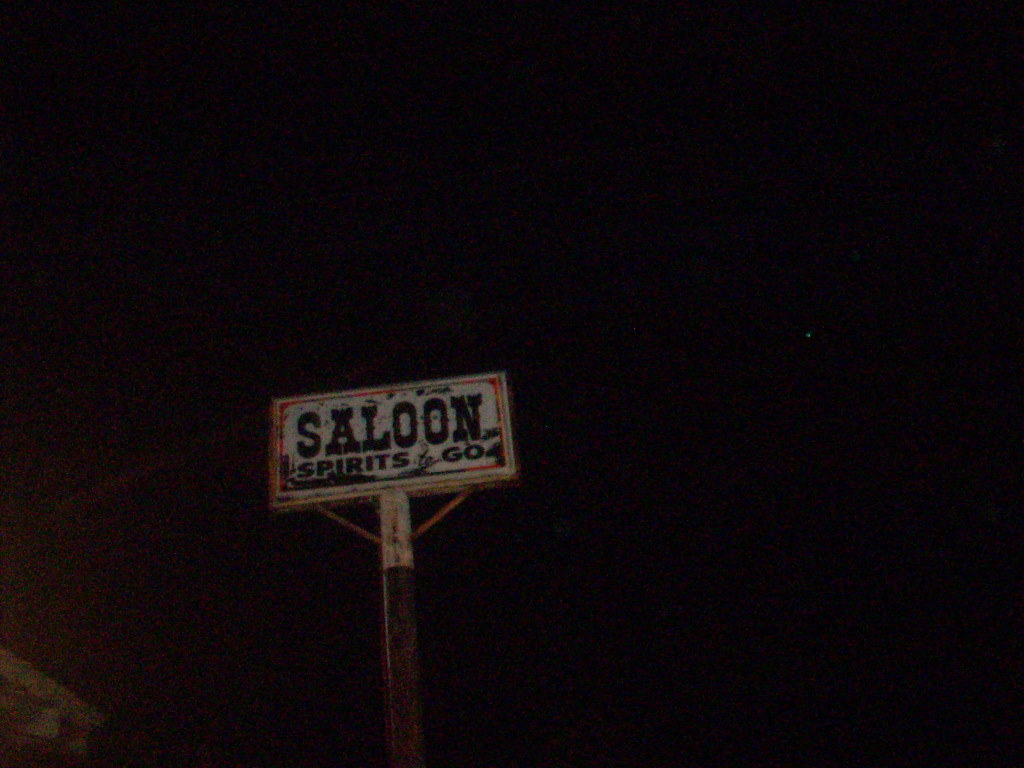The image captures a roadside sign during nighttime, set against a pitch-black background. The sign prominently features the word "Saloon" in a large, western-style black font, followed by "Spirits to Go" in a plain, smaller black font. Both phrases are displayed on a white background with a red outline bordering the sign. The sign, weathered with rust, sits atop a pole that starts white at the top and turns brown further down. To keep the sign in place, two diagonal arm pieces, resembling buttresses, extend upward from the pole. In the background, a small illuminated dot, likely a star, is visible in the black night sky. Additionally, there's noticeable red dotting throughout the pole and sign, as well as on the left side of the image, hinting at possible lighting or reflections. Intriguingly, the very corner of a building's roof is visible at the bottom left, adding a hint of context to the sign's location.